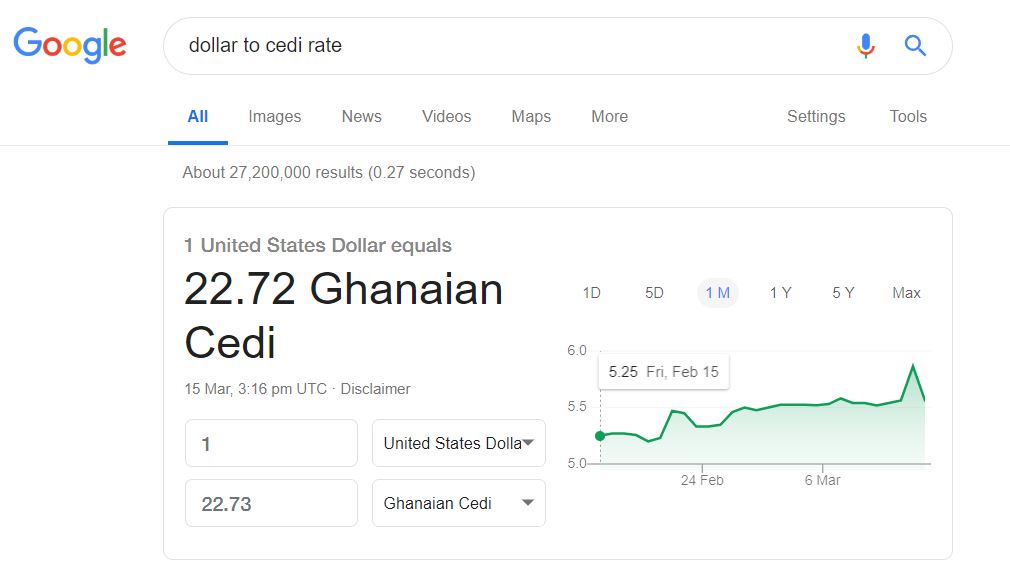The image features a Google search results page set against an all-white background. Dominating the left side of the image is the iconic Google logo, depicted in vibrant blue, red, yellow, and green lettering. Positioned to the right of the logo is a search bar containing the query "dollar to SETI rate" typed out in black letters.

To the right of the search bar, there is a blue microphone icon with a red semi-circle beneath it, and a blue magnifying glass icon next to that. Below the search bar, the word "All" appears in blue, underlined to indicate it is the selected tab, with other categories like Images, News, Videos, Map, More, Settings, and Tools displayed in light gray text.

Further down, the page informs us that there are approximately 27,227,200 results, which were generated in 0.27 seconds. This information is conveyed in very light gray lettering. 

The immediate search result states "1 United States Dollar equals 22.72 Ghanaian SETI" in bold, dark black lettering. Next to this result, the phrase "1 United States Dollar equals" is repeated in gray lettering. To the right, a graph is displayed, showing currency trends in blue and green. The graph includes various grey labels and one blue label marked "1M" at the top.